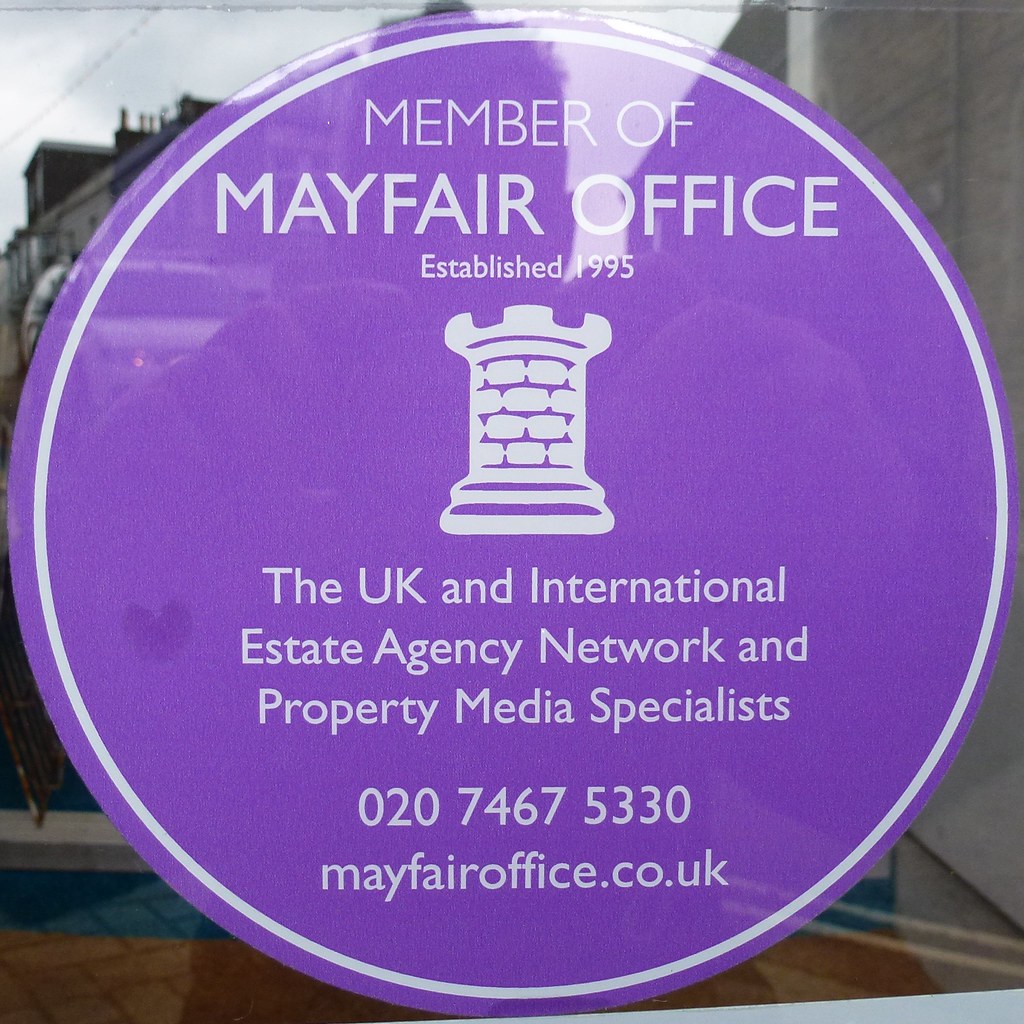The image is a color photograph featuring a circular purple advertisement sticker affixed to a glass window. The sticker consists of a purple background with a white border and white typography. At the top, it reads "Member of Mayfair Office" in bold letters, followed by "Established 1995" in smaller text. Below this is a white illustration resembling a chess piece, and further down, the text describes it as "The UK and International Estate Agency Network and Property Media Specialists." The contact details "02074675330" and "mayfairoffice.co.uk" are listed at the bottom. The window reflects various elements of the outside environment, including a building with sharp architectural points in the upper left corner, a gray sky with patches of white, and a vertical power line. Reflections on the right side reveal a gray wall, while the bottom left shows a brown floor transitioning to blue bricks with red and blue shadows. A strip of gray is visible just behind these reflections.